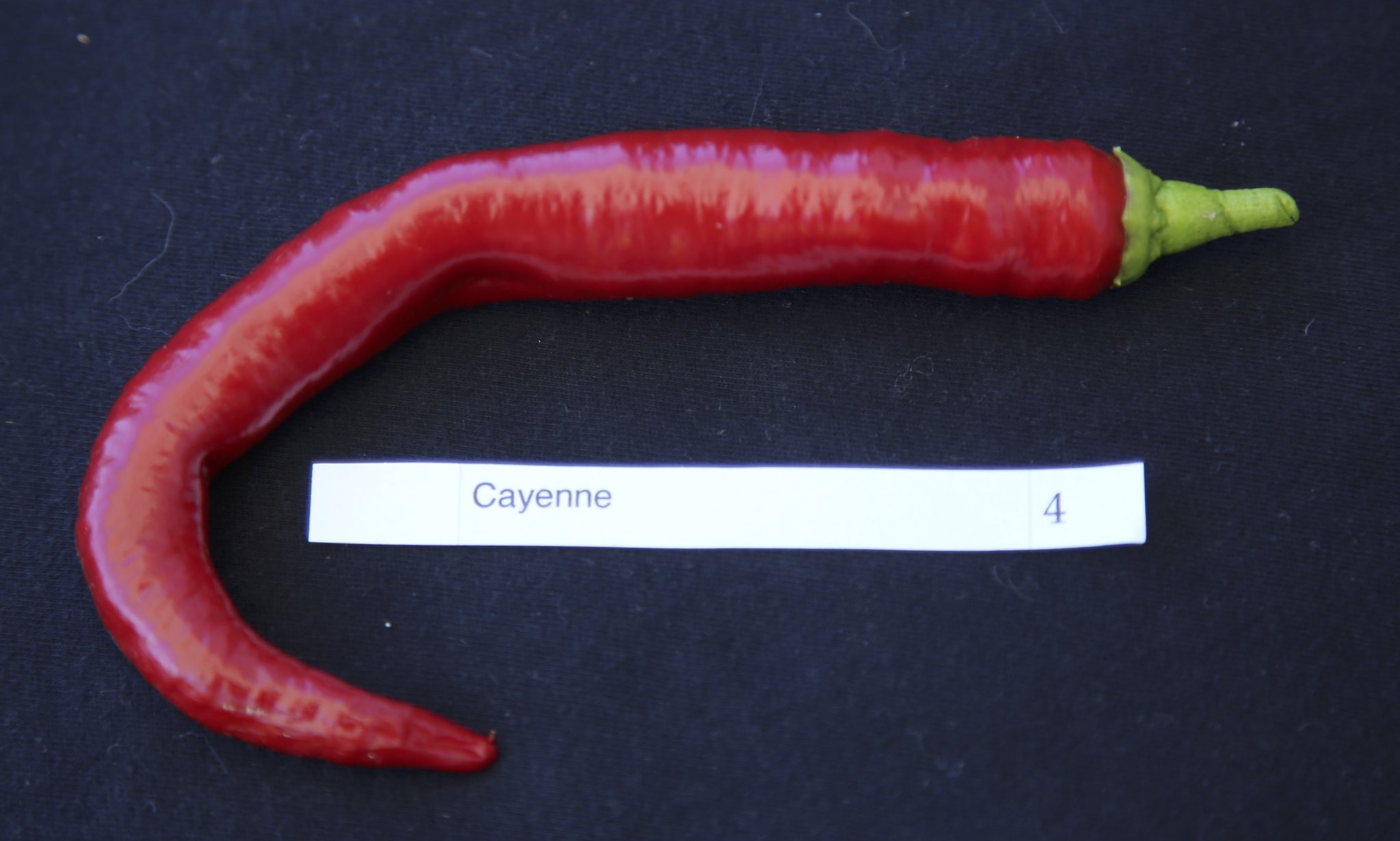The image features a bright red cayenne pepper with a green stem, positioned on a dark grey fabric background that appears slightly worn and has white lint scattered across it. The pepper has a unique hook-like, curving shape, forming a C-shape at its tail. It is shiny, with a waxy texture, and the green stem stands out prominently. Beside the pepper is a thin, white rectangular piece of paper that reads "CAYENNE" on the left side and "4" on the right side in black font. The high-quality photograph is landscape-oriented, capturing the intricate details of the pepper and the textured fabric background.